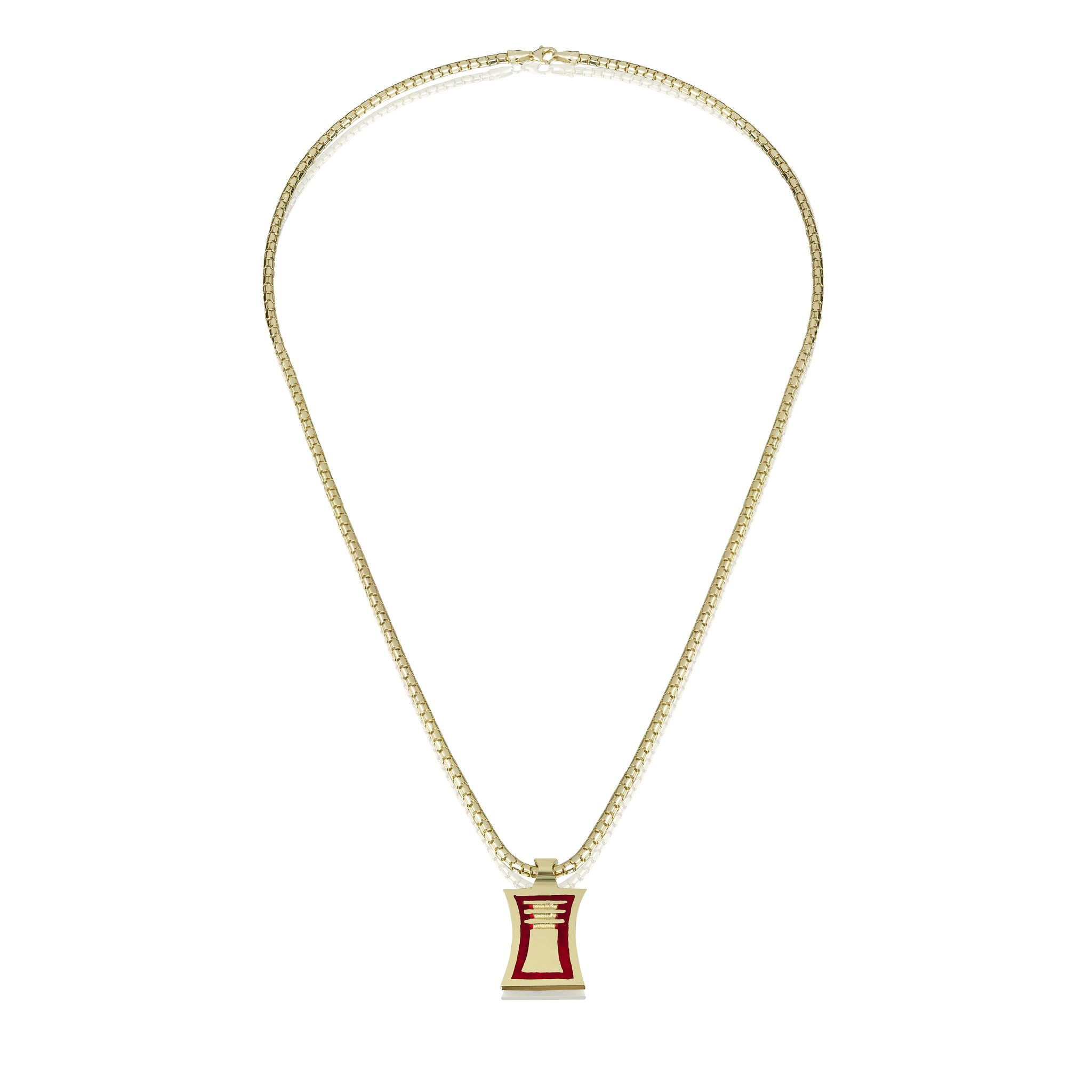This is a detailed photograph of a gold necklace, prominently displayed against a white background. The necklace features a tightly linked gold chain, resembling 14 karat gold, and is neatly clasped at the top with a lobster claw clasp. The chain is arranged in an oval shape, wide at the top and narrowing towards the bottom, almost resembling a hot air balloon. Hanging from the necklace is a distinctive gold pendant. The pendant is a square shape with concave sides, featuring a red inlay in the center. Atop this red background are three gold lines, forming a design that vaguely resembles a bell or a small, intricate structure. The pendant measures roughly half an inch in length and appears slender and elegant, possibly designed for an advertisement or catalog display. The overall presentation emphasizes the delicate craftsmanship and aesthetic appeal of the necklace and its pendant.